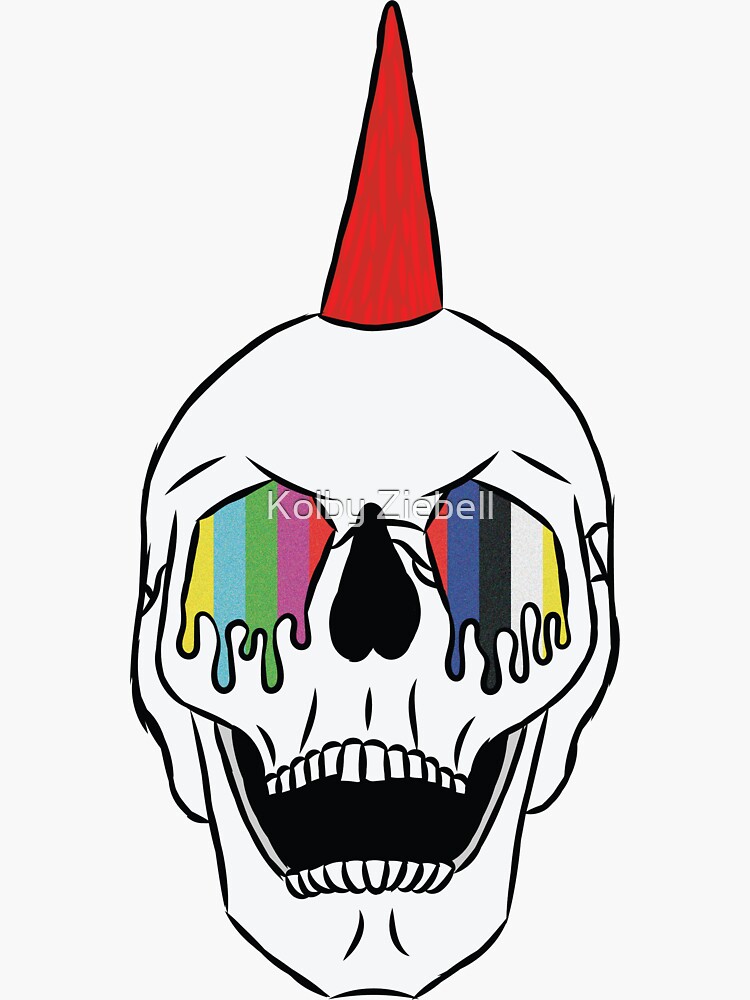This detailed illustration depicts a white skull set against a light gray background. The skull features an open mouth with visible teeth and a black interior. The nose area is black as well, resembling an upside-down narrow heart, giving the impression of a missing nose. At the top of the skull, a prominent red horn protrudes. The most striking element is the eyes, which are a vivid array of colors—yellow, light blue, green, purple, red, dark blue, black, and white—melting and dripping down like paint splatters. This creates a rainbow effect with vertical streaks. A watermark, "Cola Bell Hunt Cole," is also present in the illustration.